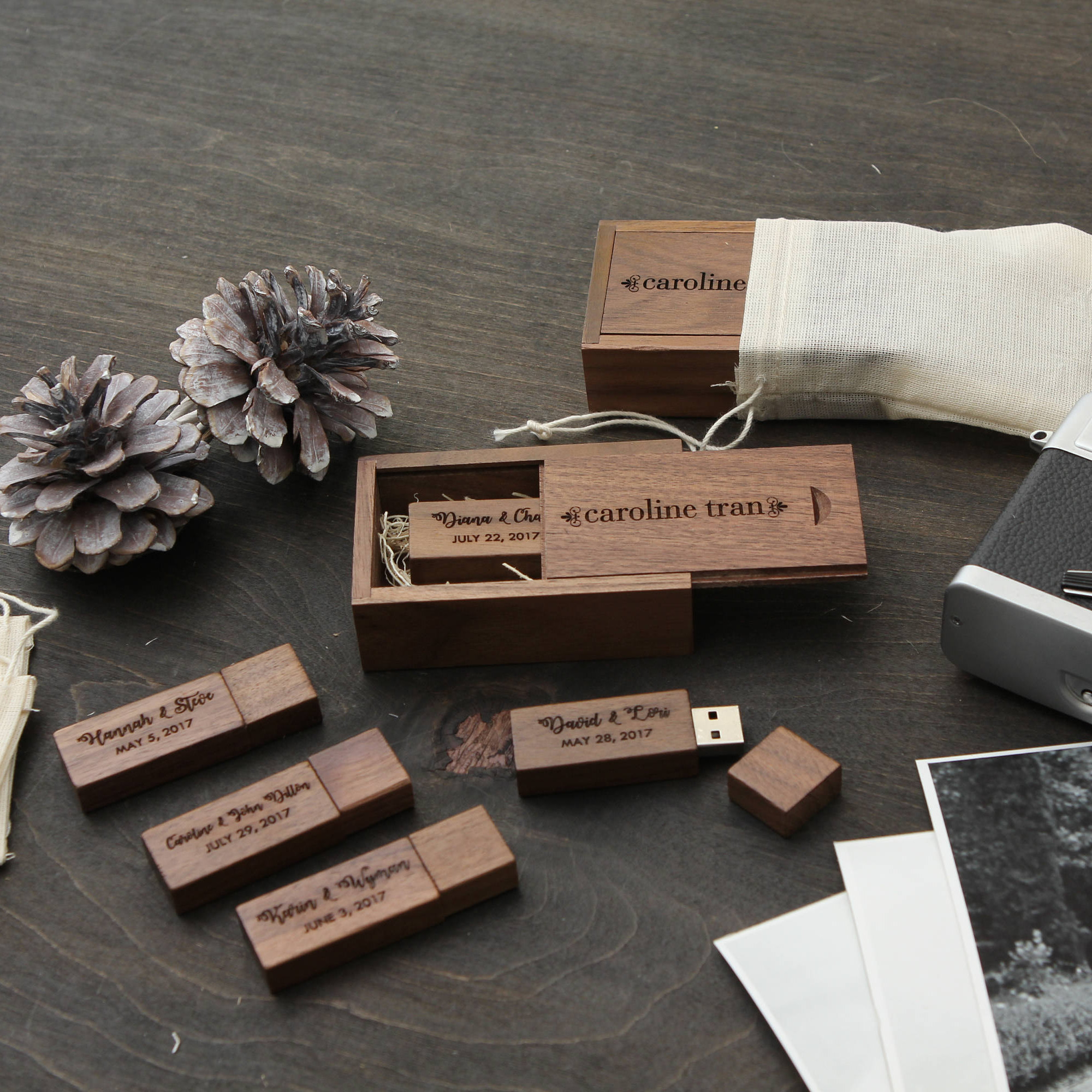The image depicts a rustic, dark wooden countertop displaying several custom-made, hand-carved, wooden USB drives each engraved with different couples' names and dates, indicating they might be wedding gifts or party favors. Surrounding these USB drives are a few small accents: two pine cones on the left, a couple of tiny canvas drawstring bags, and some black-and-white Polaroid photos peeking from the right side next to a camera. The USBs are beautifully crafted, with matching wooden caps and are nestled inside small, engraved wooden display boxes, one of which is partially open revealing a USB stick surrounded by bits of string. Engravings on the USBs include names like "David and Laurie, May 28th, 2017,” “Hannah and Steve, May 5th, 2017,” “Caroline and Julio, July 29th, 2017,” “Karen and Kevin, June 3rd, 2017,” and a partially visible “Diana, July 22nd, 2017.” This meticulously arranged setup could very well be an advertisement for an Etsy shop or similar service specializing in personalized, engraved wooden keepsakes.